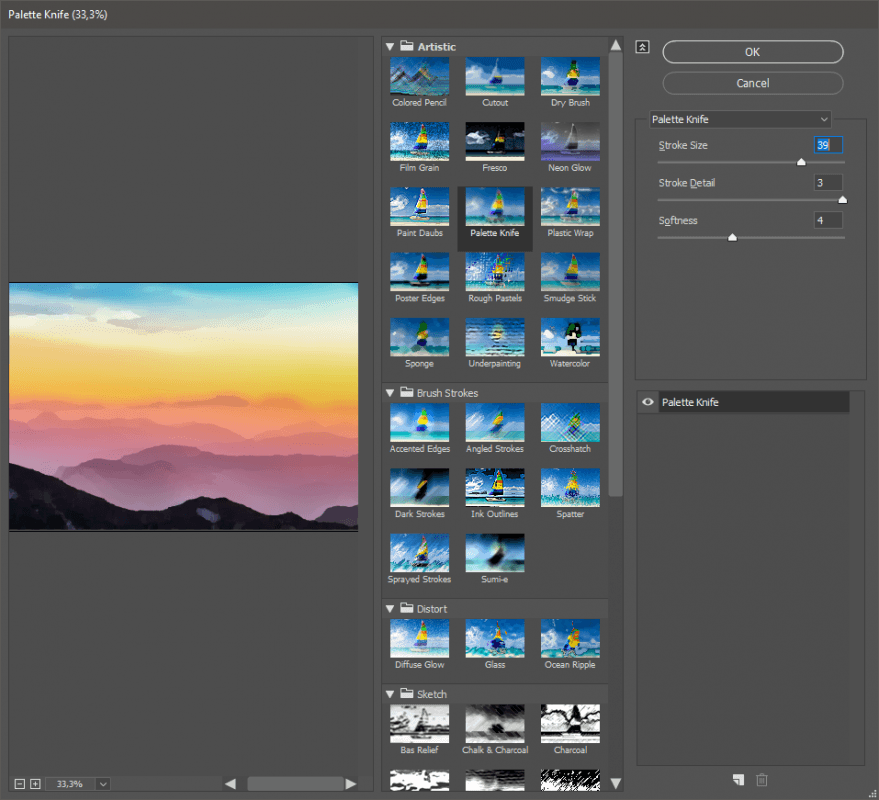In the image, a person is seen manipulating digital artwork on a laptop. The screen displays an application window titled "Palette Knife," with the zoom level set at 33.3%, likely indicating the current view percentage of the image. The artwork being edited resembles a brush-painted sunset, featuring vibrant hues of orange, pink, and hints of purple, along with a foreground showcasing mountains or valleys.

On the right side of the screen, there is a drop-down menu labeled "Artistic," containing a folder with various image manipulation options. The first set includes several sailboat images that appear to be crafted using different artistic techniques, such as colored pencil, cut-out, and dry brush. Each line in this menu displays three distinct images, and there are five lines in total for this category.

Below this, another section titled "Brush Strokes" offers various options for altering brush strokes, including accented edges, angled strokes, cross hatching, and dark strokes. Additional categories for "Distorting" and "Sketching" are also available, with the latter focusing on black-and-white effects.

At the bottom right of the screen, there are "OK" and "Cancel" buttons for applying or discarding changes. The "Palette Knife" section allows detailed customizations, where users can adjust numerical values for stroke size, stroke detail, and softness. There is also an option labeled "Palette Knife," but it currently appears to be blank.